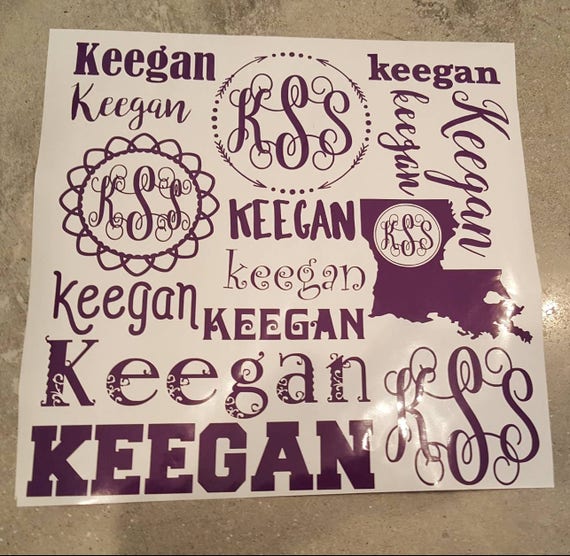The image features a detailed, off-center collage of custom-made decals set against a stone-like background with a tan, gray, and black texture. The central collage, displayed on a square sheet with an off-white background, primarily showcases the name "Keegan" in various purple fonts, including known styles like Letterman and Curls MT. The sheet also contains four distinct decals of the initials "KSS" in a stylish, curvy script font, each with unique designs: a geometric arrangement with dots and arrows, a sunburst outline, the shape of Louisiana with "KSS" in the northern part, and a standalone cursive decal in the lower right corner. The collage, appearing to be laid on a marble countertop, is illuminated from above, capturing slight glares. In total, there are 11 instances of "Keegan" and four of "KSS," giving a personalized and artistic touch to the display.